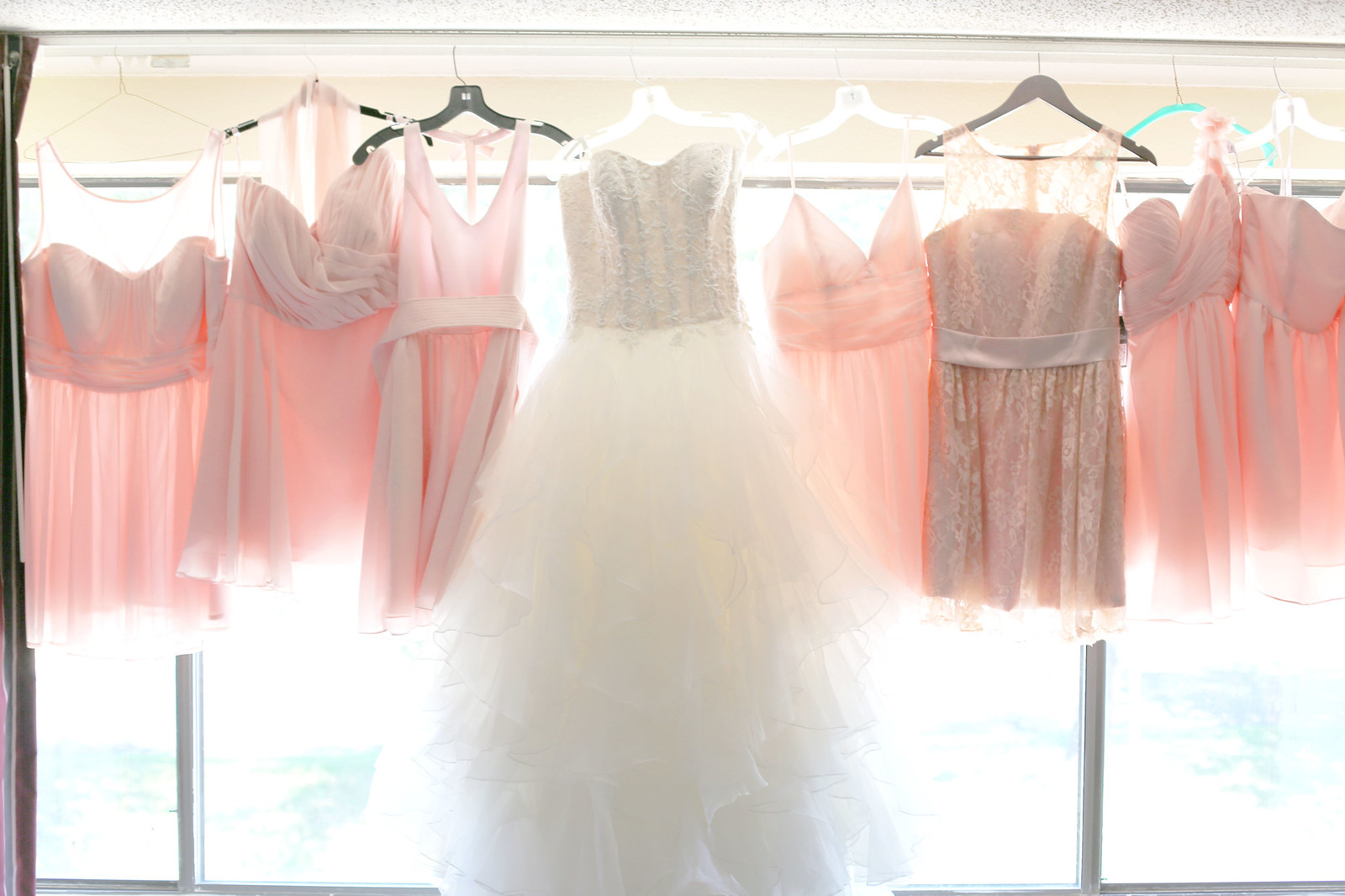A photograph captures a stunning display of a bridal and bridesmaid ensemble set against a backdrop of large windows trimmed in black metal or wood. Central to the image is an exquisite bride's wedding dress with a strapless, white satiny bodice transitioning into a long, layered tulle skirt, which shimmers softly with light streaming through. Surrounding it are the bridesmaid’s dresses, arranged on either side, hanging from black hangers attached to a pole along the ceiling. These dresses are uniformly short, fashioned in varying shades of light pink with mix of strapless and clear-strapped, V-neck tops, and delicate netting or sheer slips overlaying pink satin skirts. The whole arrangement is backed by a somewhat blurred, light-filled background, lending an airy and ethereal quality to the scene.